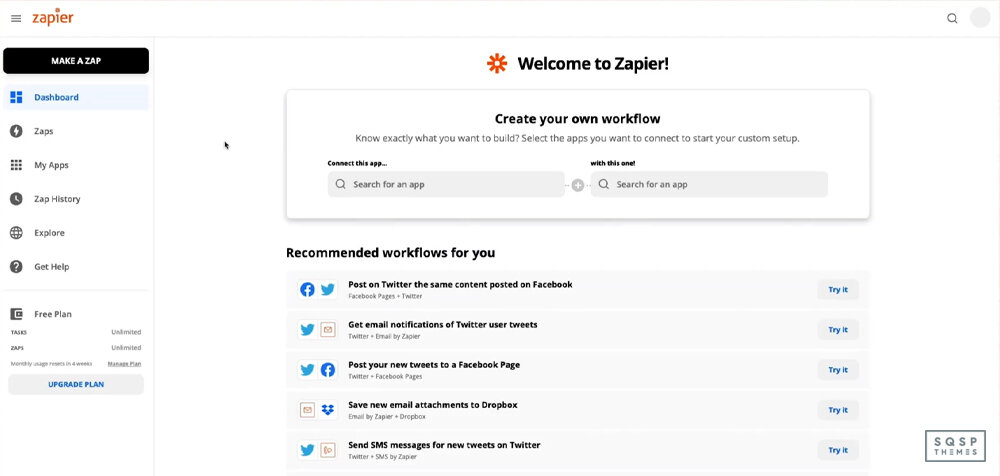The image displays the Zapier dashboard. At the top, there is a red banner with the word "Zapier" prominently displayed. On the right side of the banner, there's a magnifying glass icon indicating a search function. On the left, there's a drop-down menu. Above the banner, a black button labeled "Make a Zap" is visible, aiming to initiate the creation of a new workflow.

Beneath the banner, a navigation menu lists the following options in sequence: Dashboard, Zaps, My Apps, App History, Explore, Get Help, and Free Plan. Adjacent to these options, a gray button labeled "Upgrade Plan" invites users to enhance their subscription.

To the right, a welcome message reads, "Welcome to Zapier, Create Your Own Workflow." Instructions follow to "Know Exactly What You Want to Build," "Select the Apps You Want to Connect," and "Start Your Custom Setup." Beneath this, prompts to "Connect This App" and "With This App" each lead to corresponding search boxes for users to select the desired applications.

At the bottom, suggested workflows are listed under the heading "Recommended Workflows for You," including:
- "Post on Twitter the Same Content Posted on Facebook"
- "Get Email Notifications of Twitter User Tweets"
- "Post Your New Tweets to a Facebook Page"
- "Save Some Small Attachments to Dropbox"